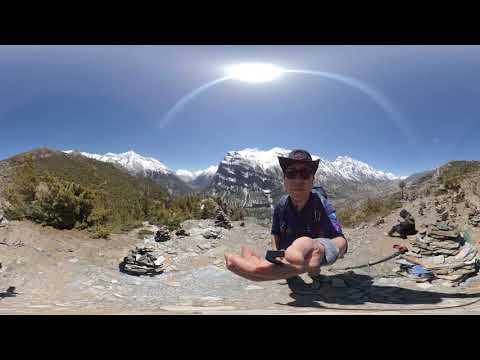The photograph showcases a highly distorted image likely captured with a fisheye lens, giving it a warped, panoramic appearance. Central to the image is a man crouched down, seemingly taking a selfie with his arm extended towards the camera, holding a black pole, possibly a selfie stick. He is looking directly at the camera with an open, upward-facing palm. The man is dressed in a short-sleeve blue button-down shirt, dark sunglasses, and a short-brimmed hat resembling a cowboy hat. The environment around him is a natural rocky landscape, featuring gray dirt and stone piles on both his left and right sides. Shrubbery is visible just behind him, leading further back to a range of snow-capped mountains under a clear blue sky with minimal clouds. The sun is shining brightly at the top center of the image, casting noticeable light streaks that curve due to the lens effect. Additionally, another figure dressed in dark colors is squatting on the right side of the photograph. This second figure further accentuates the expansive and rugged terrain, dotted with mounds of stacked stones and bordered by tall, green pine trees on the distant ridgeline.